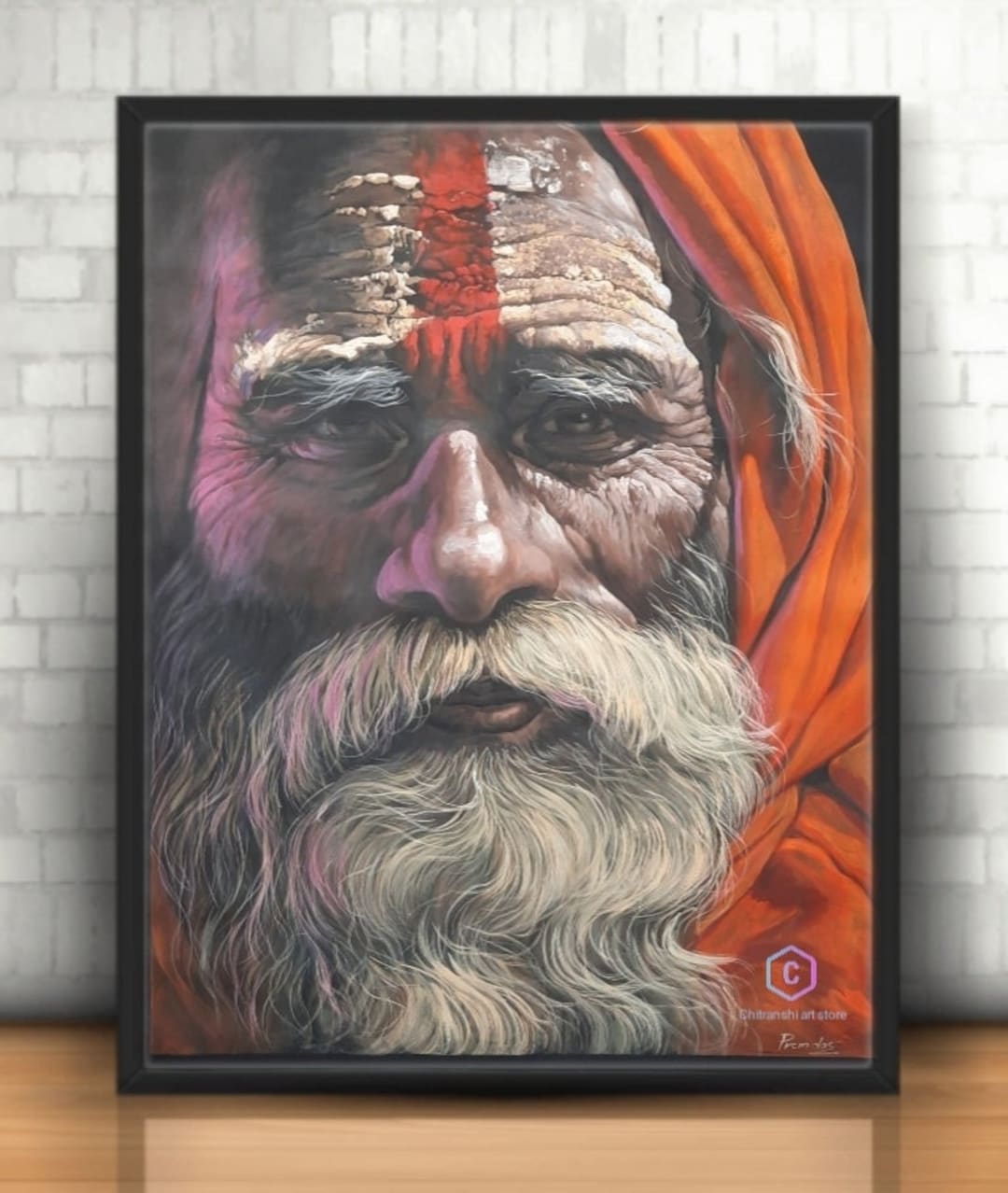In this photograph, a detailed portrait of an elderly man prominently features in the center, framed in black and set against a white brick wall with a reflective wooden floor. The man in the painting has distinctive facial features, including a large mustache and a long, white beard, accompanied by bushy eyebrows. His wrinkled face, covered in white clay or some similar substance, is further marked by a vertical red line extending from the center of his forehead. He is dressed in a saffron robe, with a hood draped over the left side of his head, reaching down to his neck and shoulders. The painting, which appears to be religious or indicative of a holy man, includes fine details such as a copyright logo at the bottom right corner, representing "Chetan Trashy Art Store." This setting, a mixture of homely and sacred vibes, showcases an image within an image, emphasizing the aged man's serene and spiritual demeanor.